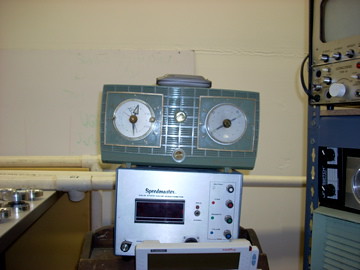The image depicts a fascinating array of vintage machinery, prominently featuring an antique green device mounted atop another silver machine. The green apparatus is accented with gold square outlines and sports two analog dials—reminiscent of old clocks—positioned on either side. A grayish cap crowns this device, adding to its mechanical intrigue. Beneath it, the silver machine has a white pipe attached, likely part of its operational mechanisms. The scene is set against an off-white, somewhat dingy wall, which hints at an industrial or workshop setting. Surrounding the main equipment, numerous control knobs and dials are scattered across various adjoining machines, indicating a complex and possibly archaic technological environment. The precise function of these machines remains unclear, evoking a sense of curiosity and mystery.